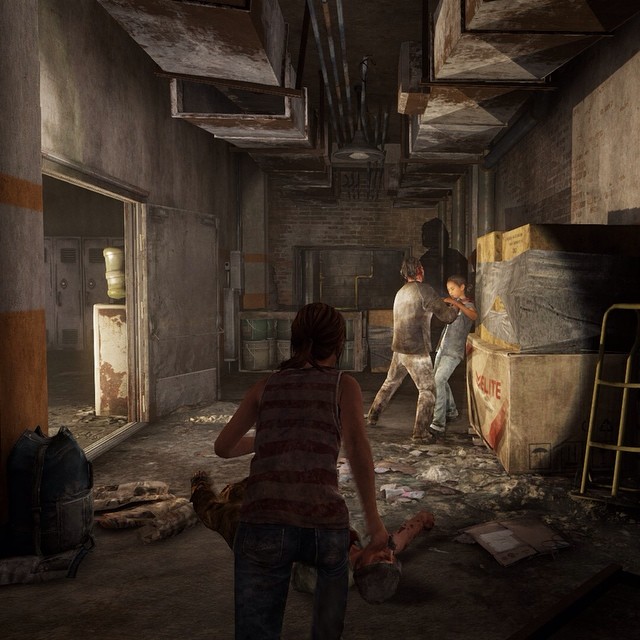In this haunting image captured inside a decrepit industrial building, three figures are depicted amidst the decay. Dominating the scene is a large male figure clad in grimy light-colored pants and a similarly dirty shirt, both tinged with shades of gray and brown, underscoring the overall filth. He holds a smaller figure, whose gender is indiscernible, pressed firmly against a crate. This smaller individual is dressed in blue jeans and a sleeveless blue top or T-shirt. Their arm is raised over the aggressor’s menacing grip in a futile defensive posture. 

Emerging from the bottom frame, another figure approaches, clad in dark pants and a striped tank top, possibly red and white. Suspended above all three characters, neglected steel-squared ductwork, broken and rusted in places, runs across the ceiling. The background is characterized by walls that portray a dirty gray hue and faded brick, with additional elements like an open doorway revealing a rusted, grimy water cooler and some rowing lockers. The entire setting speaks to a long-abandoned facility, steeped in neglect and time-worn abandonment.